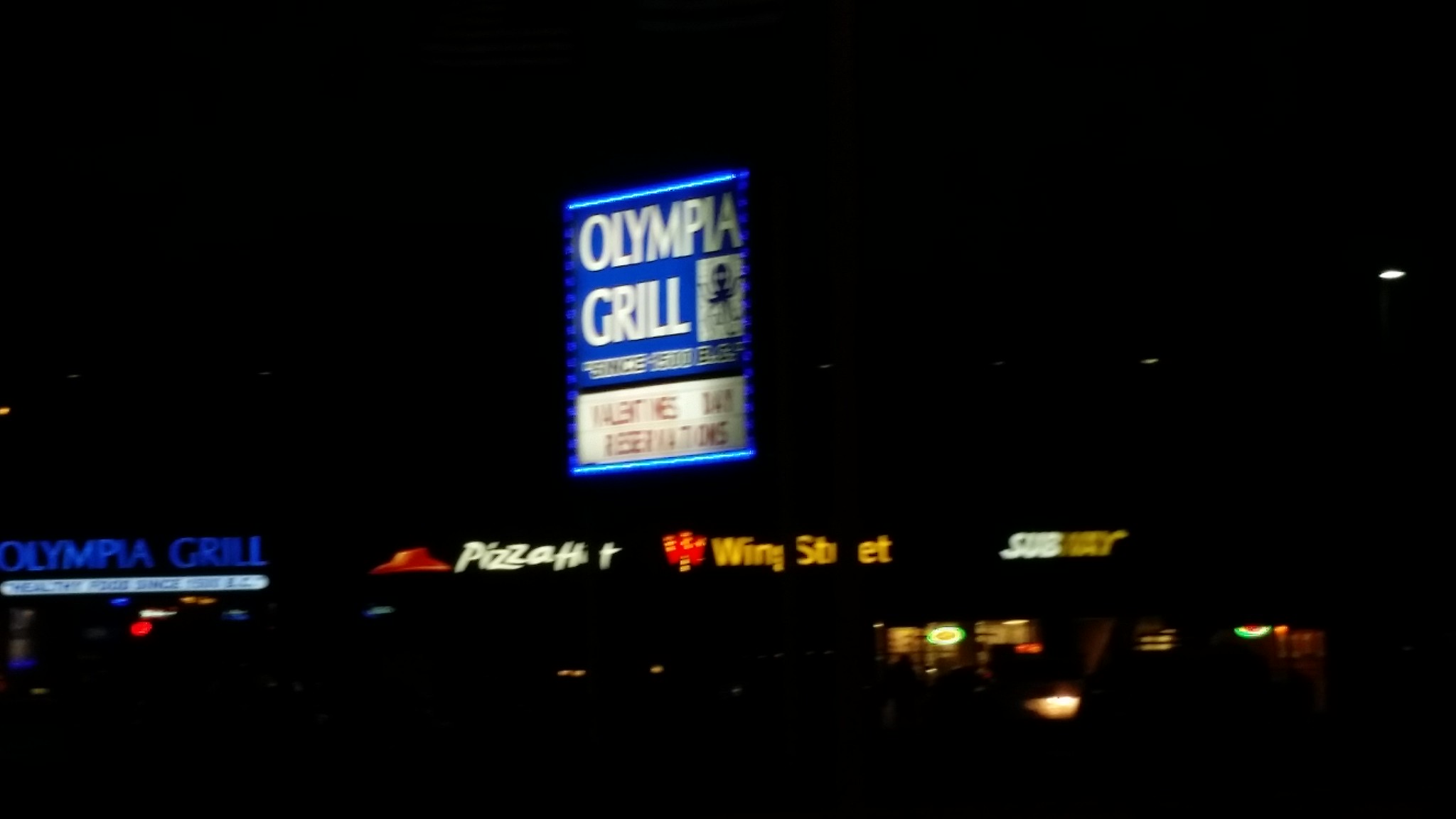The photograph captures a nighttime scene dominated by a somewhat blurry, illuminated blue sign reading "Olympia Grill" in white letters. The sign stands out sharply against the dark, black background, emphasizing the nocturnal setting. Below the primary sign, a strip mall is partially visible with a selection of establishments. The Olympia Grill sign is positioned on the left side, accompanied by a thin white line underneath. To its right, a distinctly recognizable red and white Pizza Hut sign is illuminated. Continuing to the right, a bright yellow "Wing Street" sign makes its presence known. Further along, the familiar Subway logo, with "Sub" in white and "Way" in yellow, appears lit up. Just underneath the Subway sign, a few windows with interior lights are faintly visible, contrasting against the otherwise dark surroundings. This scene encapsulates a quiet, nighttime view of a small commercial area with various dining options.